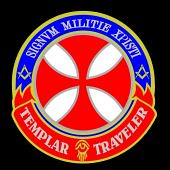The image features a logo against a solid black background. The design includes a circular medallion at the forefront, adorned with blue and red banners at the top and bottom, each outlined in gold. The top banner reads "SIGNVMMILITIEXPISTL," while the bottom banner states "Templar Traveler." In the center of the circle is a four-petal flower motif in white. The image itself is pixelated and of low quality, suggesting it may be a screenshot of a screenshot. The overall design appears to be a logo, possibly related to a soccer team or a group with a name that resembles "Sigmund Malate Kubles" and references Templar Knights.